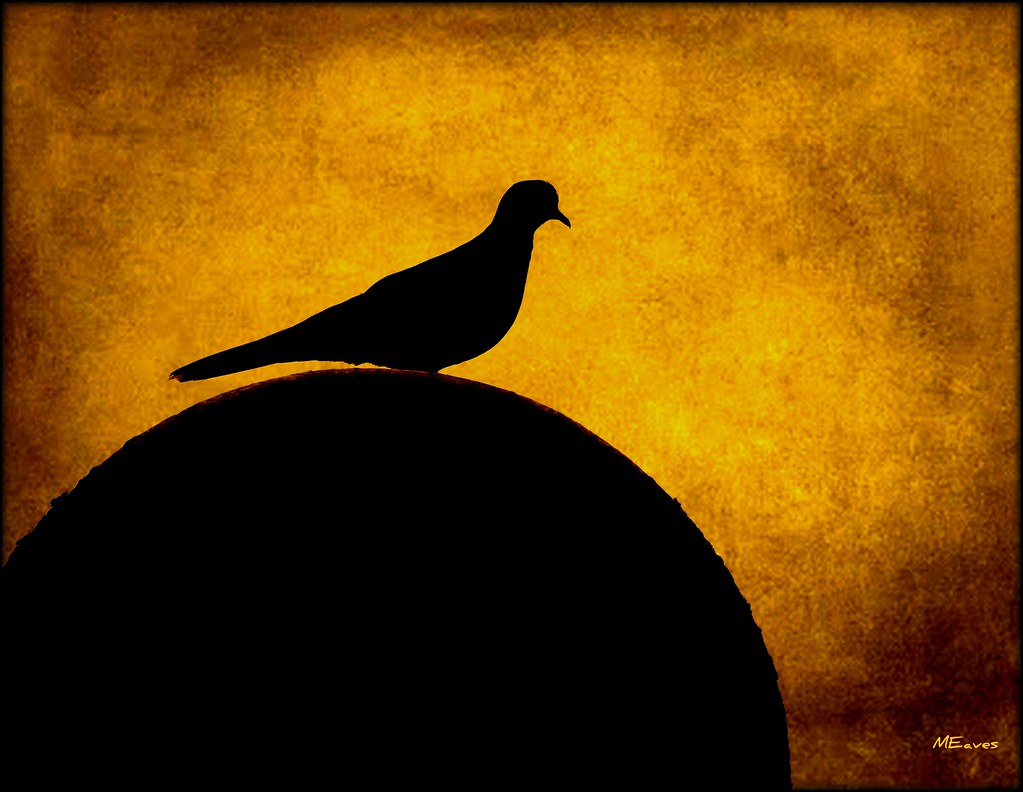This image showcases an intriguing drawing, characterized by a striking use of shadows and sepia tones. Dominating the composition, a silhouette of a dog stands out clearly. The dog's shadow is perfectly outlined against a circular element, whose exact nature—be it a sphere, a ball, or another object casting the shadow—remains ambiguous. The backdrop features a textured sepia tone, reminiscent of antique parchment or a coffee-stained surface, adding to the artwork's nostalgic and mysterious aura. In the bottom right corner, the piece is signed by the artist, lending a personal touch to this captivating visual narrative.